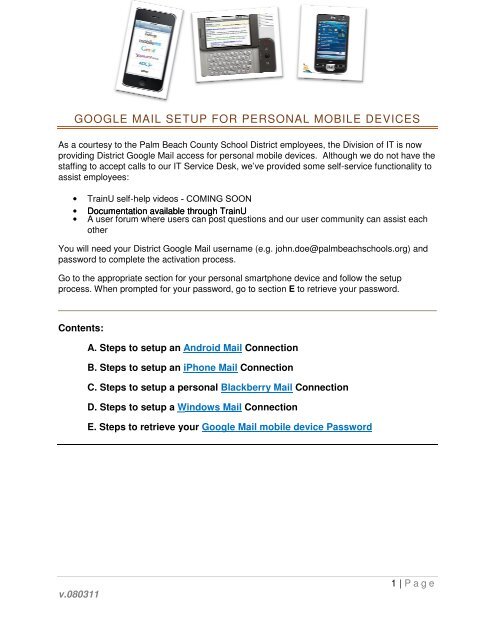The image displays a page providing detailed instructions for setting up Google Mail on various personal mobile devices, specifically aimed at Palm Beach County School District employees. At the top of the screen, the document features images of old mobile phones, including Android, iPhone, and Blackberry, highlighting its dated nature. The title, prominently displayed, reads "Google Mail Setup for Personal Mobile Devices." As a courtesy from the Division of IT, employees are informed that while direct support calls cannot be accommodated due to staffing limitations, self-service functionalities and step-by-step instructions (labeled A through E) are available to assist in setting up district Google Mail. Essential details include the requirement for a district Google Mail username and password to complete the activation process. The document is rich in text, depicting symbols and instructions aimed at guiding users through the setup efficiently.